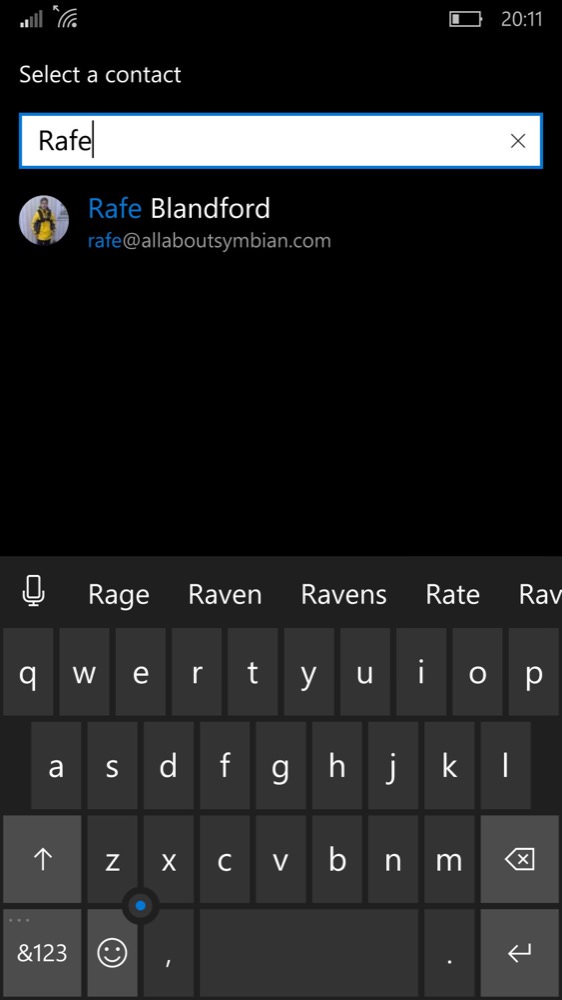The image displays a cell phone screen with a solid black background, showcasing several key elements. The cellphone's status indicators reveal low signal bars for both cellular and Wi-Fi networks, alongside a battery icon indicating nearly 20% remaining charge. The date displayed is 2011.

At the top of the screen, the text "Select Contact" is prominent. Below this, a white rectangular selection bar, bordered in blue, contains the name "RAFE," with the cursor blinking at the end of the name. Adjacent to this bar, an "X" button is positioned for clearing the selection.

Further down, the contact information for RAFE Blanford is shown. His name appears twice: "RAFE Blanford," with "RAFE" in blue and "Blanford" in white, as well as his email—"RAFE@allaboutsymbian.com"—where "RAFE" is highlighted in blue. Accompanying this information is a small circular icon featuring a photo of RAFE wearing a yellow jacket against a black background.

The lower portion of the screen displays a virtual keyboard, predominantly gray with white keys. Above the keyboard, spelling suggestions related to "RAFE"—such as "rage," "ravens," "ray," "raven," "rate," and "rave"—are listed. The keyboard includes all standard characters and has a unique blue button situated between the "Z" and "X" keys, positioned above the emoji icon. The purpose of this blue button is unclear.